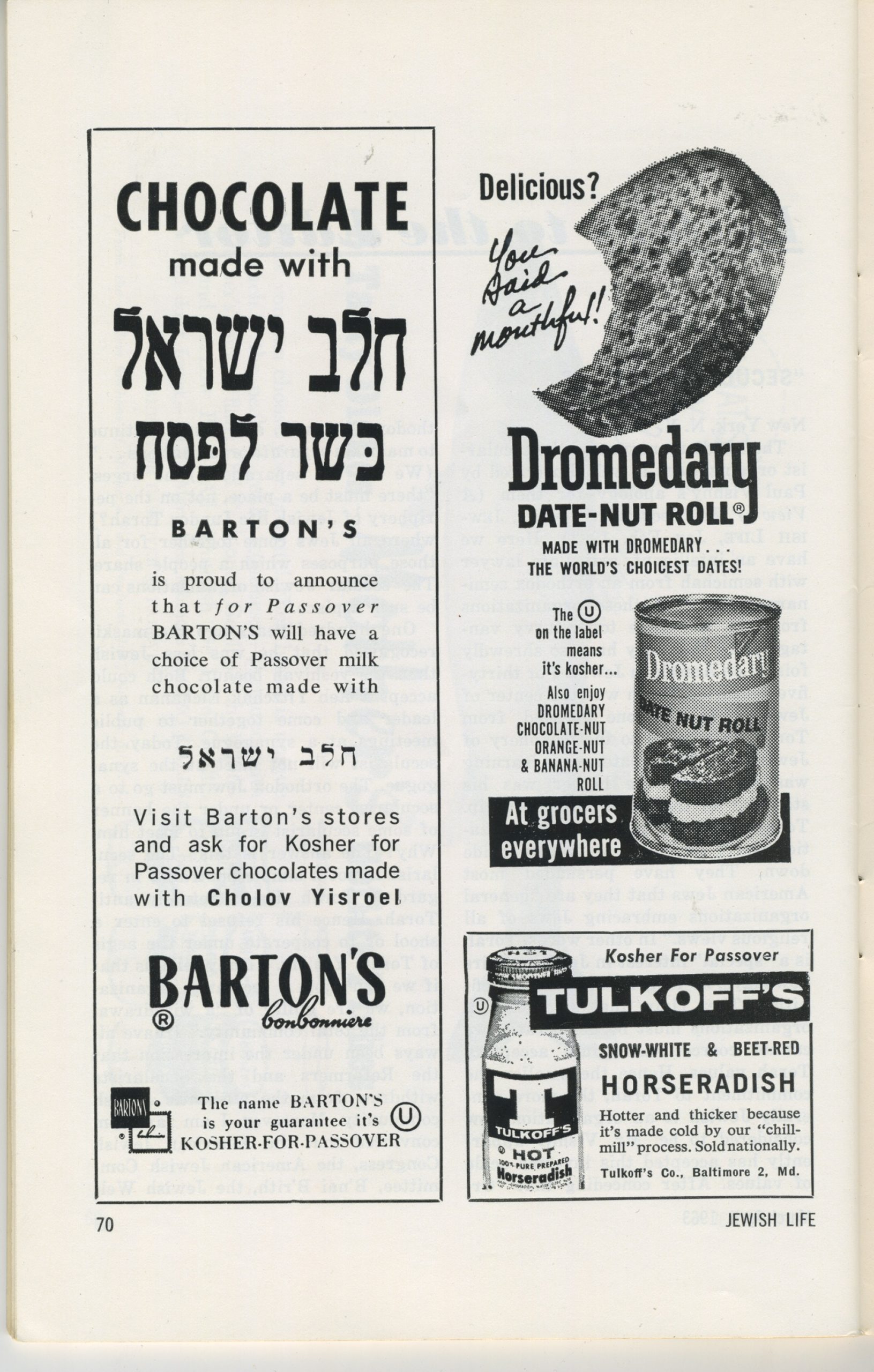This is an aged magazine page that has turned brownish over time, likely from the 50s or 60s, featuring advertisements tailored for Jewish life, indicated by the mention of "Jewish life" on the bottom right and "page 70" on the bottom left. The page showcases three prominent ads: 

1. **Barton's Kosher for Passover Chocolates**: Located on the left half, this ad proudly announces Barton's kosher milk chocolates for Passover, with text incorporating Hebrew or Aramaic characters. It encourages readers to visit Barton's stores to purchase these chocolates.

2. **Dromedary Date Nut Roll**: Positioned on the right side, this ad illustrates a can of a delectable date nut roll, described as having a bite missing to emphasize its deliciousness.

3. **Snow White and Beet Red Horseradish**: Also on the right side, this ad features a bottle of horseradish, marked as kosher for Passover, and highlights its contrasting snow-white and beet-red varieties. 

The black text stands out against the now-pale yellowish page, with the layout being a rectangle taller than it is wide, reflecting the vintage style of a classic magazine ad page filled with various grocery products.